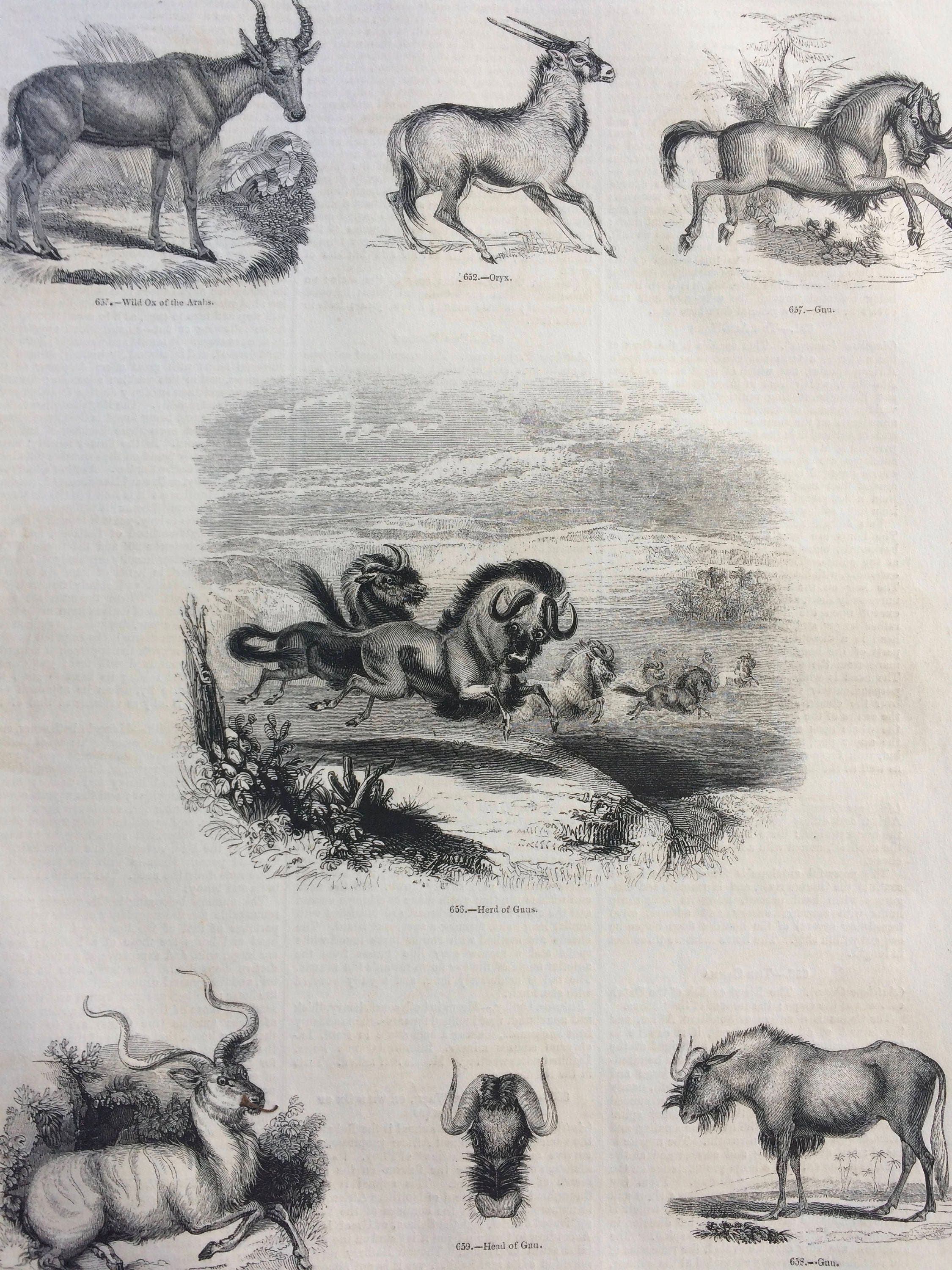This detailed black and white pencil or charcoal drawing presents a vertically rectangular scene featuring various horned animals depicted across three tiers. The upper section shows three different animals: one resembling an ox, another an Oryx with straight, pointy horns, and a third identified as a GNU, which is more horse-like with visible ears. The center of the drawing features a dynamic image of water buffaloes, characterized by their large, curled horns, energetically running and jumping over a small creek. Finally, the lower portion of the artwork presents three more horned animals: one displays S-shaped horns resembling those of an elk or gazelle, another faces the viewer head-on resembling a buffalo, while the last one shows a profile view of a buffalo, directing its gaze towards the center. The entire composition is set against a backdrop of varying shades of gray, bringing the vibrant motion and diverse forms of these majestic creatures to life.